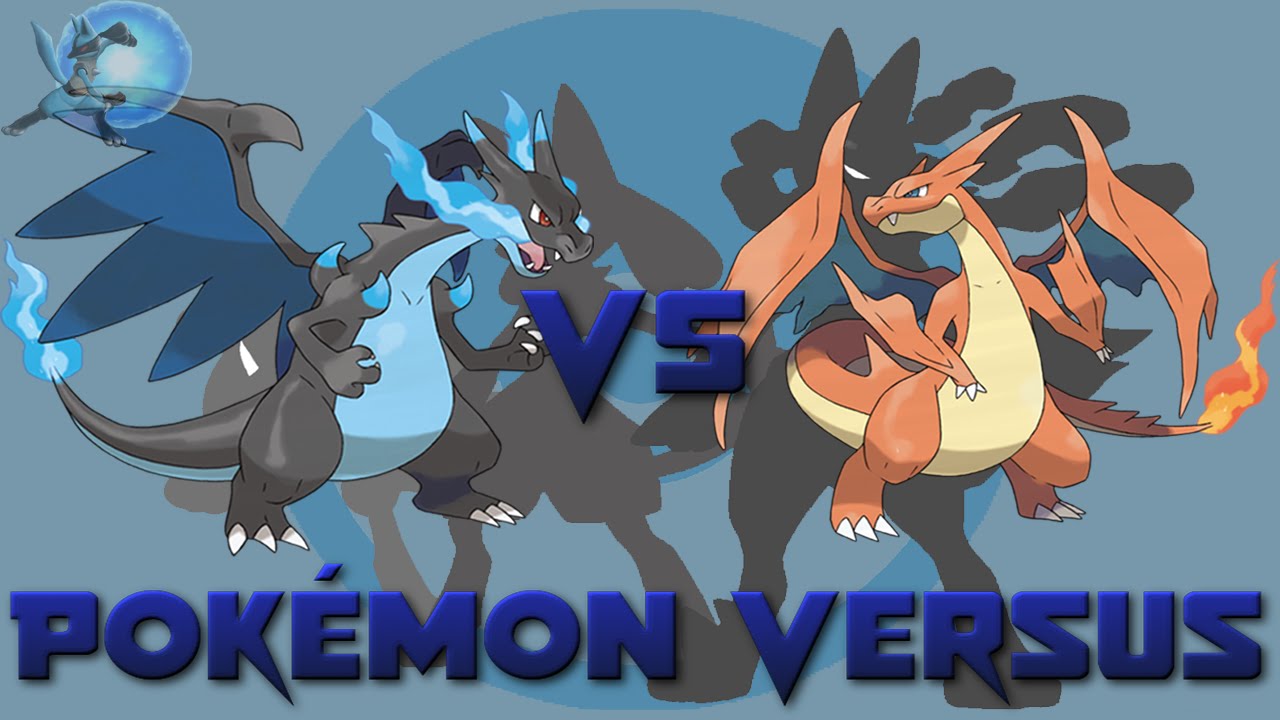The image is a vividly colored drawing, reminiscent of a poster, depicting an intense showdown between two dragon-like Pokemon. At the center, large dark blue letters spell out "VS," while the bottom of the image features the phrase "Pokemon Versus" in similarly striking blue font. 

On the left side, a dragon creature with a predominantly gray body is highlighted by blue flames emanating from its tail and mouth. Its wings are a dark blue-gray, and it has a chest and underbelly of light blue. The creature also sports red eyes and blue horns above its arms, adding to its fierce appearance. 

Opposing it on the right is a dragon with an orange body and a pale, cream-colored underbelly. This creature has orangish-yellow flames issuing from its tail and sharp fangs visible, completing its menacing look. The background subtly features shadows of additional Pokemon, adding depth to the scene. A small Pokemon in the upper left corner holds a blue bubble, contributing to the detailed composition of the artwork. Both dragon-like creatures, reminiscent of T-Rex dinosaurs with dragon heads, are locked in an aggressive staring contest, ready to clash in a fiery battle.